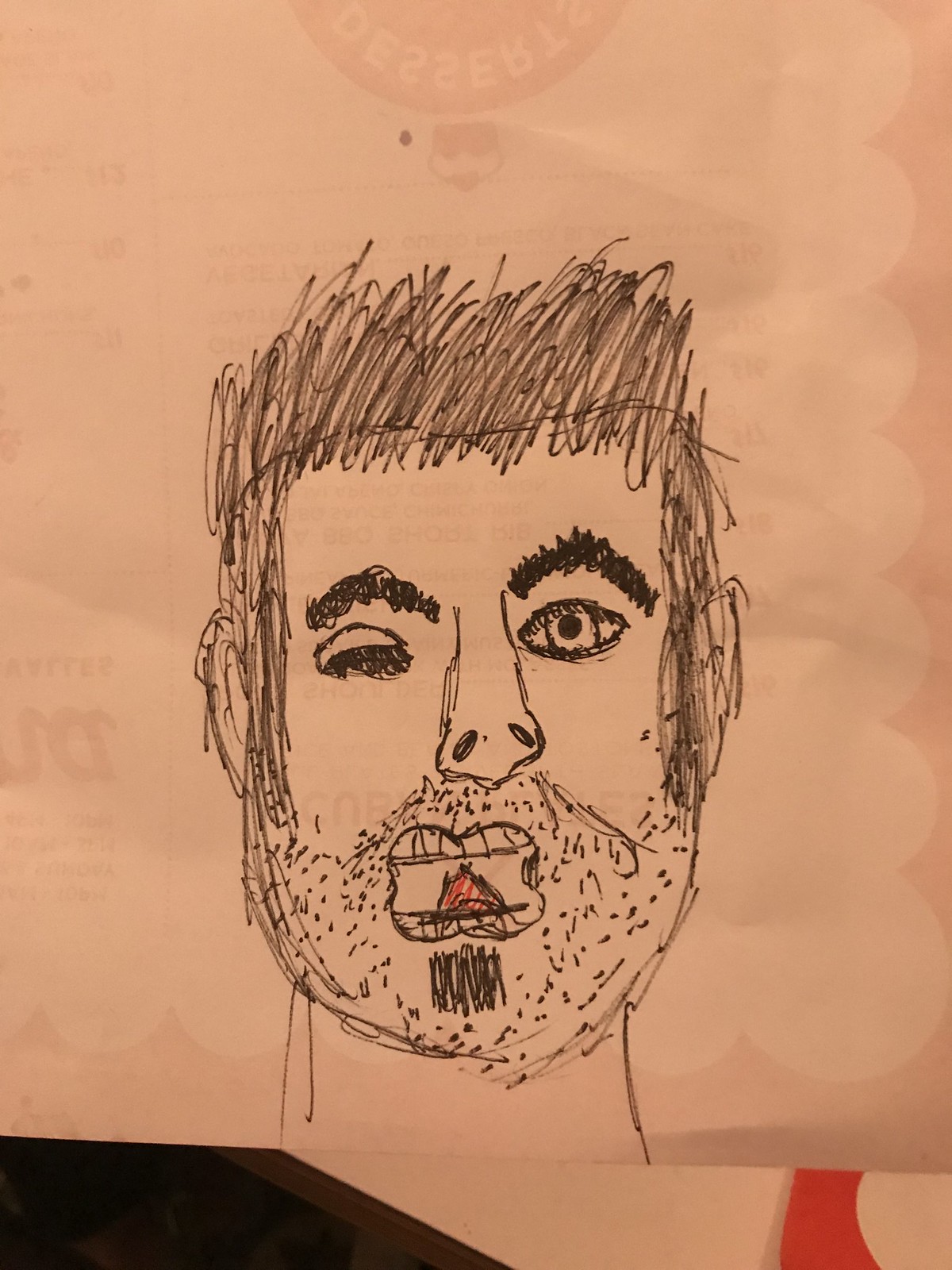A detailed pen and ink sketch captures the visage of an individual sporting a short beard. The drawing, rendered on a piece of off-white paper that resembles the texture of a shopping bag, focuses on the subject's face from the neck up. The sketch prominently features one fully open eye while the other is slightly closed, giving a nuanced expression to the portrait. The nose and bushy eyebrows are meticulously detailed, and the hair is depicted with shorter sides and longer, textured locks on top that transition into sideburns.

The mouth is open, revealing a carefully illustrated tongue with slight red accents adding a touch of color to the predominantly black ink illustration. The beard is a notable element—full yet trimmed short—with an additional detail of a slightly more pronounced goatee area beneath the bottom lip. This artist's sketch is executed with fine precision, using very fine black ink lines that intricately define each facial feature and give the piece a realistic yet expressive quality.